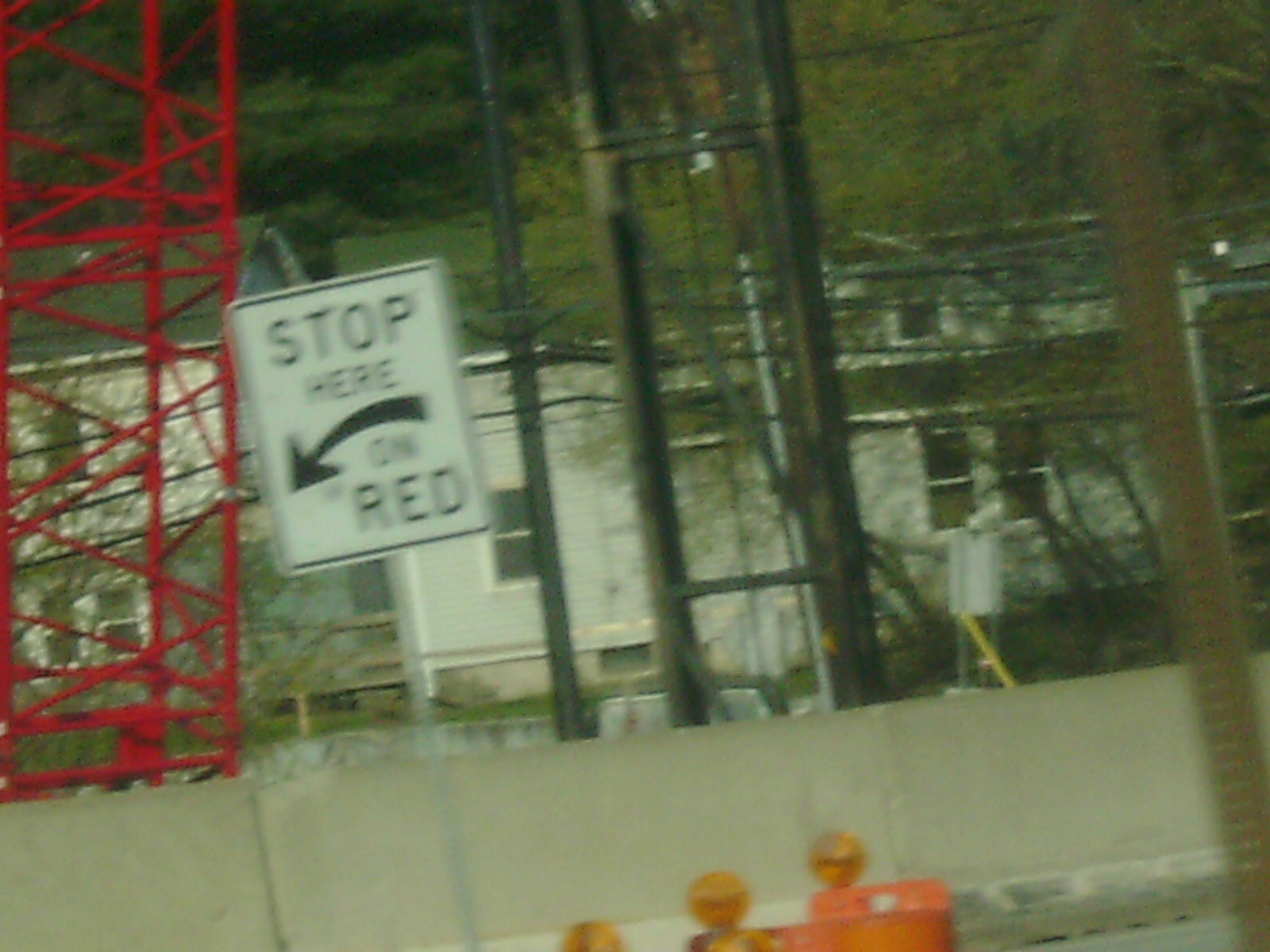A blurry and dimly lit outdoor photograph captures the perimeter of a construction zone. In the foreground, the tops of three bright orange construction barrels topped with yellow caution lights stand prominently. Just behind these, a solid cement barrier marks the boundary of the work area. Further into the scene, the skeletal frame of a red crane and the structure of a towering construct made of brown and black metal rises, signifying ongoing development. Beyond the construction zone, a cluster of residential buildings emerges in the background. A "Stop Here on Red" street sign, featuring white text on a black background and an arrow pointing to the left, is also visible. In the far distance, several trees dot the horizon, completing the layered landscape of the scene.